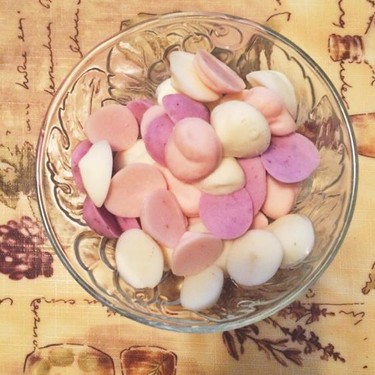In the center of this squared image, a clear glass bowl with an ornate, scalloped design holds a multitude of small, dome-shaped objects. These objects are likely candy melts, fragments of chocolate, or colorful candies, featuring shades of white, pink, light pink, dark pink, purple, light brown, and possibly pale orange. The bowl sits on a beige tablecloth adorned with hand-drawn sketches of plants, leaves, and dark cursive text, enhancing the setting's homely aesthetic. The photo is taken from above, providing a top-down view of the intricate contents and detailed background, possibly in a kitchen or dining area.